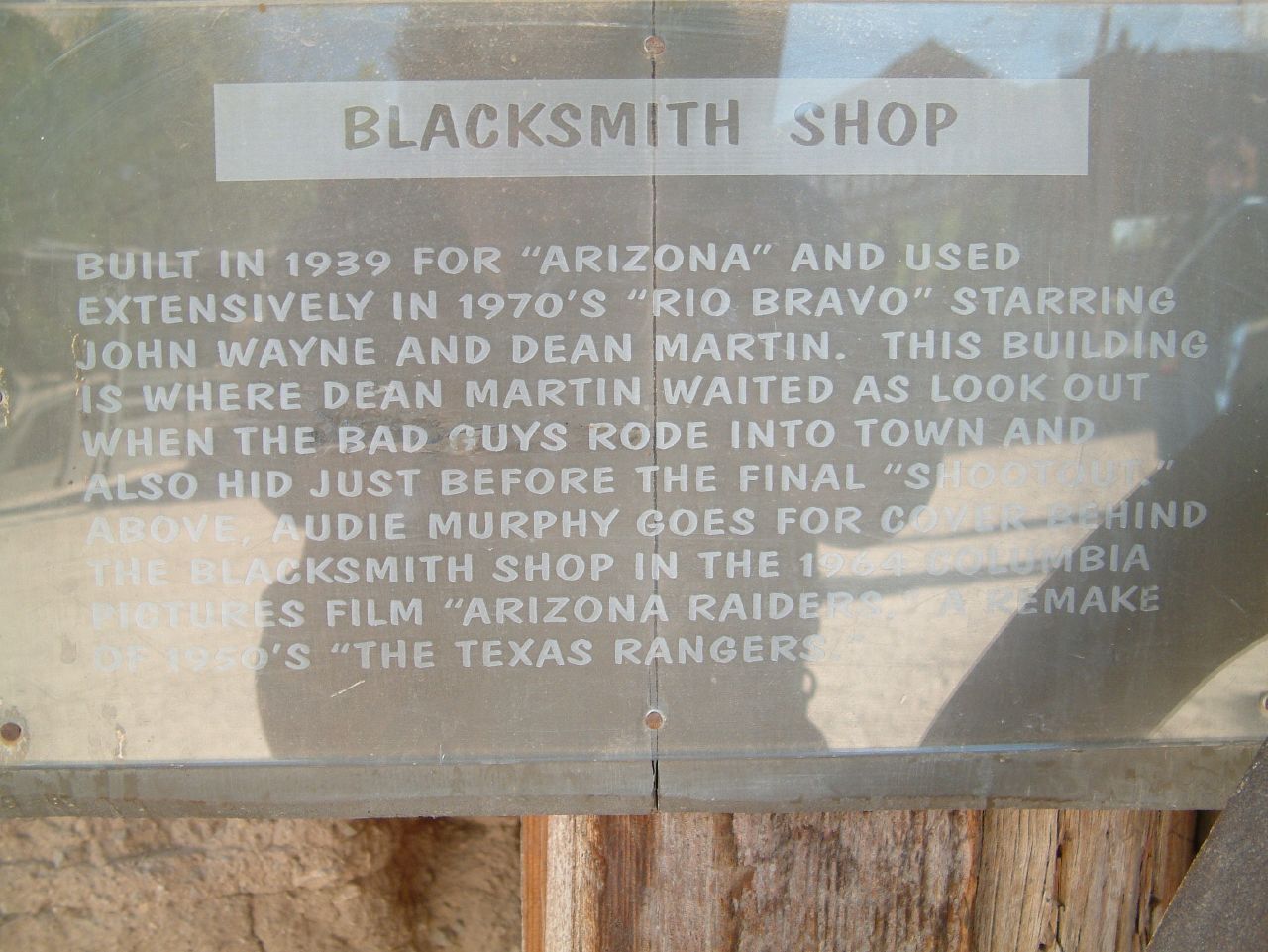The image features a detailed information plaque attached to the side of a building made of both wood and stone. The plaque, protected by plexiglass which reflects the camera person, is set against a wooden background and prominently displays the title "Blacksmith Shop" in a white rectangular box. The text beneath reads: "Built in 1939 for Arizona and used extensively in the 1970s Rio Bravo, starring John Wayne and Dean Martin. This building served as the lookout point for Dean Martin when the bad guys rode into town and was also his hiding spot before the final shootout." Additionally, it mentions "Audie Murphy taking cover behind the Blacksmith Shop in the 1964 Columbia Pictures film Arizona Raiders, a remake of The Texas Rangers." The historical and cinematic significance of the building is clearly indicated on the sign, emphasizing its role in classic Western films.